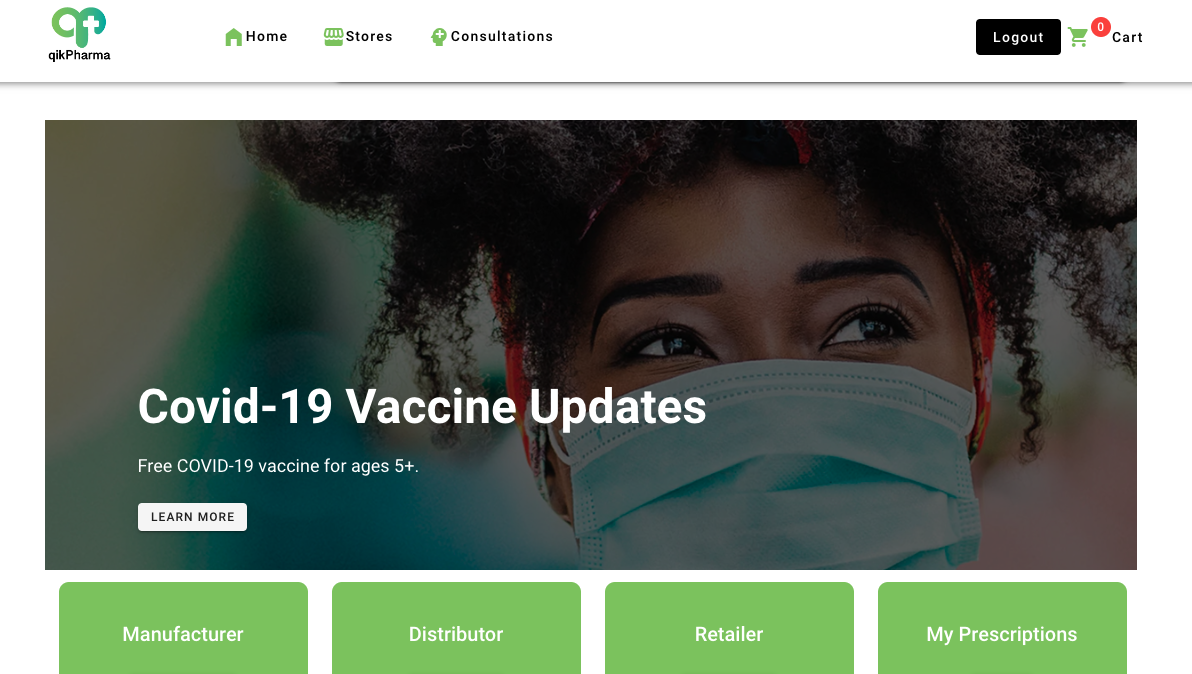The image is a screenshot from a website. At the very top of the page, there are three navigation options: "Home," "Stores," and "Consultations." To the right of these options, there is a black "Logout" button. Adjacent to the "Logout" button is a green shopping cart icon, which shows a red box with the number "0," indicating there are no items in the cart.

Below this navigation bar, there is a banner announcing "COVID-19 vaccine updates." The message highlights that a free COVID vaccine is available for individuals aged five and up, accompanied by a call-to-action button in a white box that reads "Learn More." The background of this announcement features a close-up image of a woman with curly hair wearing a face mask.

Further down the page, there are four green boxes labeled "Manufacturer," "Distributor," "Realtor," and "My Prescriptions." 

In the top left corner of the page, the company's name and logo are displayed as "Quick Pharma."